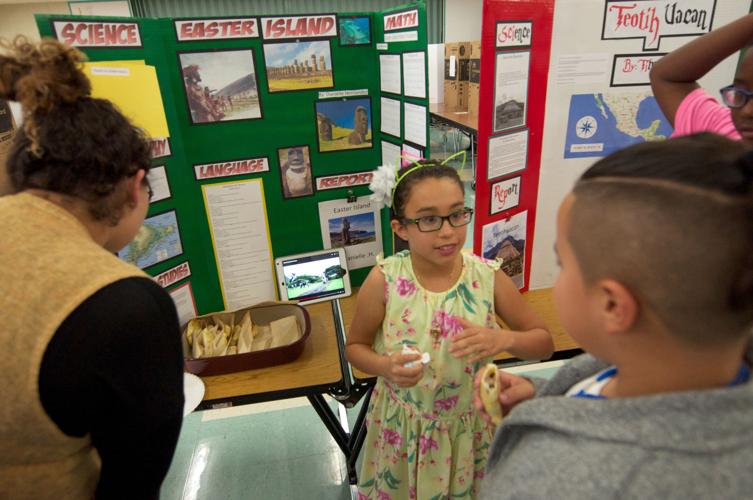In this indoor photograph, we see a bustling school event centered around a young girl in a light yellow, floral dress adorned with pink flowers and green leaves. The girl, with her hair pulled back, wears glasses and a distinctive green headband with hollow cat ears. She stands in front of a table, holding something white in her right hand, and is engaged in conversation with a young boy. To her left, an adult woman is focused on the table, which has a tray with various food items. Behind the table, a display featuring banners and posters about science, Easter Island, math, and language is prominently visible. These posters and maps suggest an exhibition related to historical monuments and statues, lending an educational atmosphere to the event. Additional banners and posters are also visible along the sides, enhancing the scholarly setting.